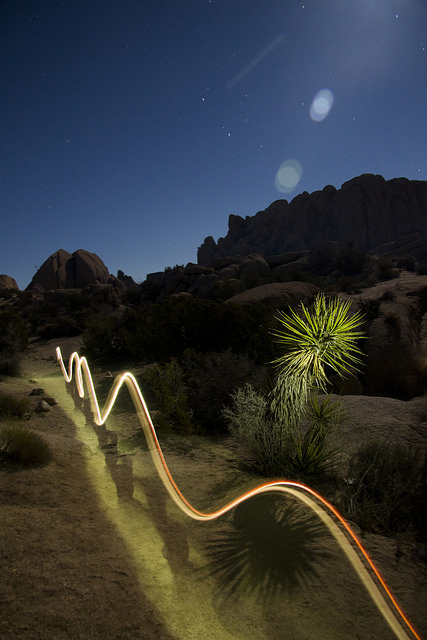In this nighttime desert landscape, the sky transitions from a deep blue near the horizon to almost black at the top, sprinkled with a few stars. The scenery features a couple of dark, dirt-brown hills or mountains, creating a rugged backdrop. The ground is sandy, dotted with various shrubs and a couple of prominent plants, including a large green plant reminiscent of a dandelion and a spiky-leaved cactus. The scene is enhanced by a long-exposure effect, capturing a wavy line of light that appears to dance through the desert floor. This illuminated loop, with hues of yellow, orange, and beige, not only traces a path through the valley but also casts a spotlight on the surrounding vegetation, including the aforementioned plants. The undulating light adds a dynamic and surreal element to the otherwise desolate and serene desert night.